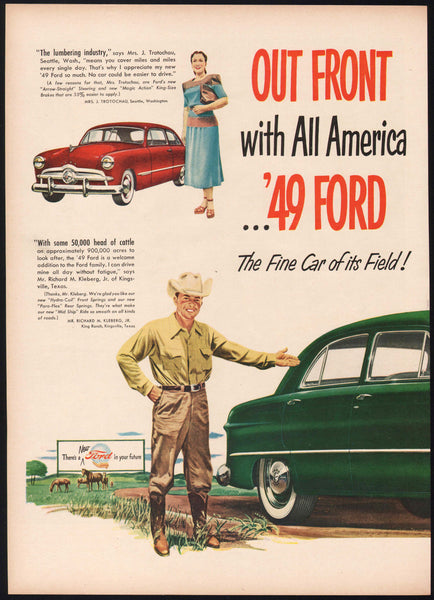This vintage advertisement for the 1949 Ford showcases a vibrant, outdoor scene with two main images. The top portion features a woman in a blue dress, holding a white purse and wearing red shoes, standing proudly next to a gleaming red Ford car. The headline above her reads, "Out front of all America, '49 Ford, the fine car of its field." Complementary text highlights a testimonial from Mrs. Trudy Show of Seattle, Washington, praising the 1949 Ford for its ease of driving and reliability over long distances, supported by phrases alluding to advanced features such as hydrocoil front springs and magic action mechanisms.

Below, the scene shifts to a rugged man in a green shirt, brown pants, brown boots, and a cowboy hat, pointing toward a green Ford car. This part of the ad emphasizes the durability and comfort of the Ford, even for demanding tasks like managing a vast ranch. A testimonial from Mr. Richard M. Kingsburg of Kingsville, Texas, underscores the vehicle's capability and comfort, making it an essential part of his daily operations overseeing 50,000 head of cattle and 900,000 acres. The billboard in the background reinforces the message with the phrase, "There's a new Ford in your future," and a pastoral scene with horses grazing completes this nostalgic look into the Ford's storied past.